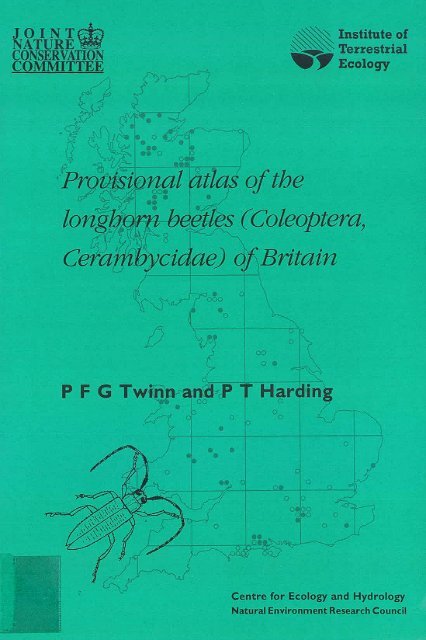The cover of this Provisional Atlas of the Longhorn Beetles (Coleoptera: Cerambycidae) of Britain is a bright green book, showcasing an intricate and scientific rendering of a beetle at its center, accompanied by a background map of Britain marked with black and white dots indicating the beetles' locations. At the top left, the text "Joint Nature Conservation Committee" is written in black, while the top right corner displays the logo and name of the "Institute of Terrestrial Ecology". The monochrome logo appears as a road splitting into two. The title spans the middle, reading "Provisional Atlas of the Longhorn Beetles Coleoptera: Cerambycidae of Britain", flanked by the authors' names, P. F. G. Twin and P. T. Harding. The bottom right corner contains the text "Centre for Ecology and Hydrology, Natural Environment Research Council". Overall, the cover combines meticulous scientific illustration with formal institutional logos and titles, all rendered in black ink on a vibrant green background.